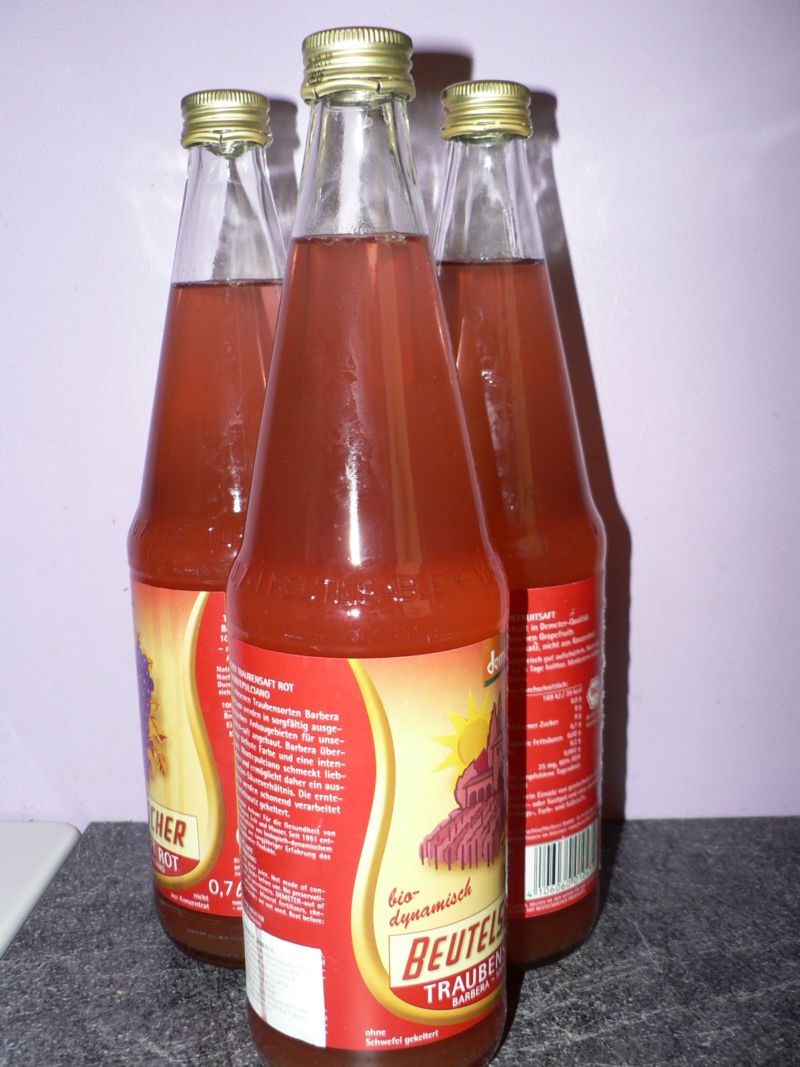This photograph features three identical glass bottles containing a light pinkish-red liquid, likely a grape-based beverage. The bottles are made of clear glass and are topped with golden metal screw caps. Each bottle bears a label, predominantly red and yellow with white text that is not in English. The legible text includes the words "Biodynamisch", "Beutels", and a partially visible "Trojben", which suggests a connection to grapes. The bottles have a cylindrical body that tapers conically towards the top, which gives them a sleek, elegant shape. They are arranged in a triangular formation on a gray marble countertop, with one bottle in the front and two behind it, casting shadows on the white wall in the background. The labels feature intricate designs, including what appears to be a large pyramid motif, adding an artistic flair to the presentation. The text on the labels, though largely illegible, suggests a biodynamic origin, hinting at a finely crafted, possibly artisanal beverage. The lighting in the photograph highlights the clarity of the glass and the vibrant color of the liquid, creating a visually appealing and detailed presentation.